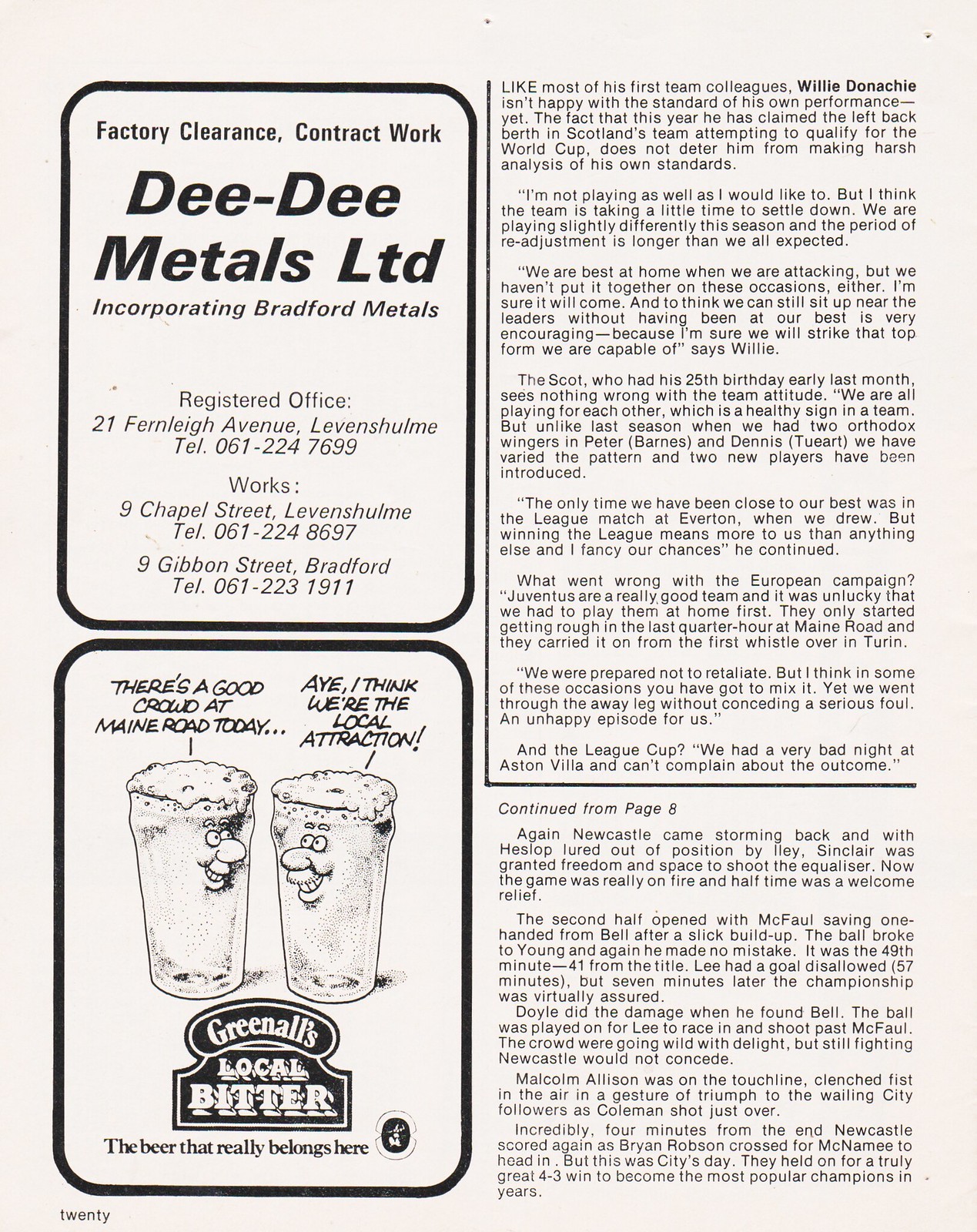This image depicts a page from a printed catalog or magazine, divided into four sections, with significant emphasis on the left quadrant. At the top left, there is an advertisement for DD Metals Ltd, which incorporates Bradford Metals. The ad lists the registered office at 21 Fernlay Avenue, Lavenshulme, with a contact number of 061-224-7699, all in black font. Directly below, occupying the lower left quadrant, is a playful ad for Greenall's Local Bitter featuring a comic drawing of two beer glasses conversing. One says, "There's a good crowd at Main Road today," to which the other responds, "I think we're the local attraction," both glasses depicted smiling. The page is identified as the 20th, with a continuation of articles on the right side. The overall color scheme includes black and white tones, with the clear, printed text and illustrations conveying a vintage, newspaper-like style.